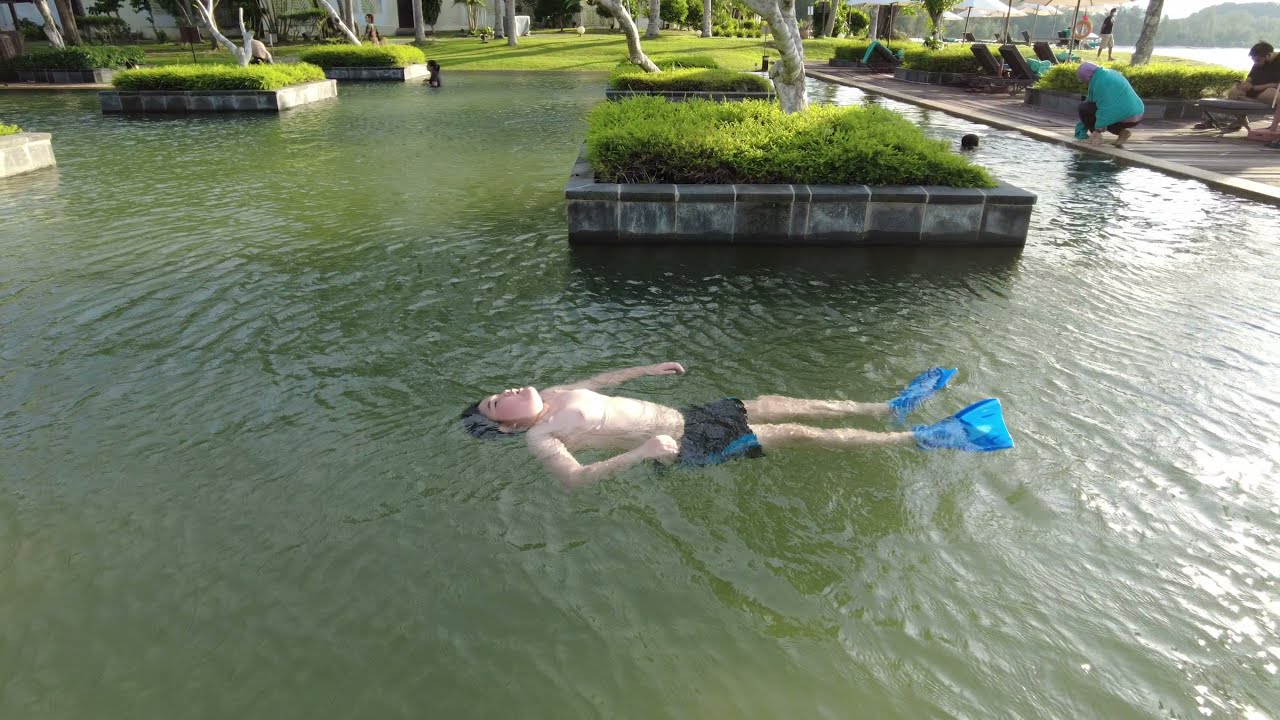The image captures a large, man-made fountain area, reminiscent of the sizeable urban water features often found in city squares. In the center of the fountain, a boy is lying on his back, floating peacefully in black swim trunks adorned with blue stripes and wearing blue swim fins. The waterbody is dotted with several concrete square planters containing lush green grass and small trees, adding a touch of nature to the geometric arrangement. 

The background reveals a grassy lawn area accompanied by buildings, suggesting the presence of a park or urban space. Towards the right of the image, a person in a green coat is seen walking away on a sidewalk, leading up and to the left. Further back, other individuals are meandering on the grassy expanse, with some lounge chairs visible, setting a scene of relaxed outdoor activity.

In the upper right corner of the image, the outline of a distant body of water and rolling hills add depth to the landscape. Notably, near the water’s edge, a woman in a blue jacket kneels on a wooden boardwalk, accompanied by a seated man, subtly integrating human presence and tranquility into the vibrant outdoor context.